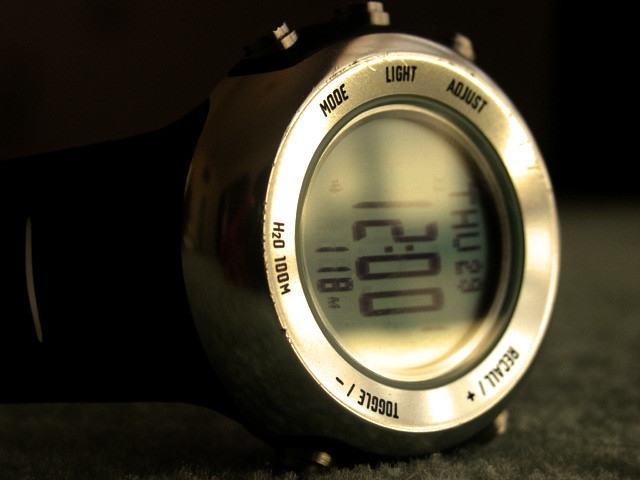The image is an up-close, detailed photograph of a thick, round, digital watch with a silver rim. The watch is positioned on a dark, carpeted surface, illuminated solely by its own light, giving the background a nearly black appearance. The watch face displays the day as "Thursday 29th," the time as "12:00," and an additional readout showing "118M," possibly indicating depth or another time zone. Around the perimeter of the watch, there are several labeled buttons in black text, including "Mode," "Light," "Adjust," and a "Toggle." Notably, the text also mentions "H2O" and "100 meters," indicating that the watch is waterproof to 100 meters. The close-up shot reveals the watch’s worn condition with visible chips and a highly reflective silver surface. This antique-like, multifunctional watch suggests robust features typical of a high-powered, possibly underwater timepiece.